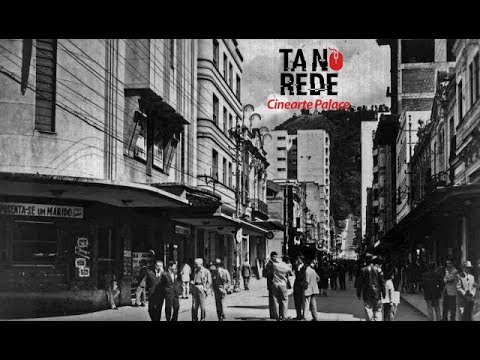In this vintage black and white photograph, likely from the 1940s or 1950s and possibly depicting a busy street in Chicago or New York, the cityscape unfolds in remarkable detail. The image is framed by tall buildings lining both sides of the street, creating an almost tunnel-like appearance, with windows arrayed along their facades. In the top center of the photo, there is a logo reading "Tan Reed" with what appears to be the silhouette of a computer mouse next to the 'N', and below this logo, the words "Sanarte Palace" are prominently displayed in red. The street is alive with activity; numerous pedestrians, predominantly men dressed in suits with some even wearing hats, walk with their hands in their pockets. On the corner of the street, a small shop with a large window showcases several posters decorating its walls. Above the street, electrical lines crisscross, adding to the urban landscape. In the distant background, the street recedes into shadows, where tall multi-story buildings are visible, and the sky frames the scene, hinting at either greenery or a hazy, indistinct horizon.